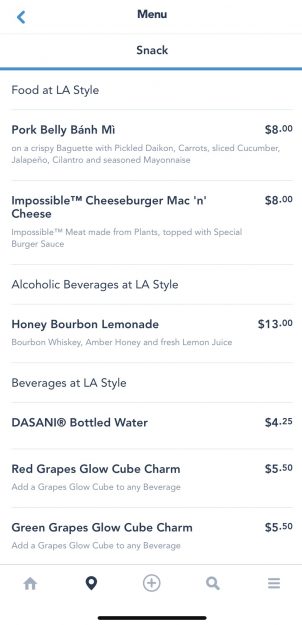Here is your cleaned-up and detailed descriptive caption:

"This is a cell phone screenshot of a menu with a white background. At the very top, there's a white rectangle subtly edged in light gray. Within this rectangle, on the left side, there's a bright blue arrow pointing left, resembling a sideways "V" in the center. The word 'Menu' is prominently displayed in bold black text. Below the word 'Menu' is a horizontal gray line.

Further down the menu, about three lines below, the bold black heading 'Snack' appears, followed by a solid blue line running horizontally across the screen. Below this line, on the left side and in gray text, is the header 'Food at LA Style' with the actual menu items listed in rectangles beneath it.

The first menu item is 'Pork Belly Banh Mi,' which is bolded in black and priced at $8.00, with the price listed to the right. The next item is 'Impossible™ Cheeseburger Mac and Cheese,' also bolded in black and priced at $8.00.

Following these food items, there is a section titled 'Alcoholic Beverages at LA Style,' underlined by a horizontal line. The first item in this section is 'Honey Bourbon Lemonade,' priced at $13.00. Below this, under a section titled 'Beverages at LA Style,' the menu lists 'Dasani Bottled Water' for $4.25, 'Red Grapes Glow Cube Charm' for $5.50, and 'Green Grapes Glow Cube Charm,' also priced at $5.50."